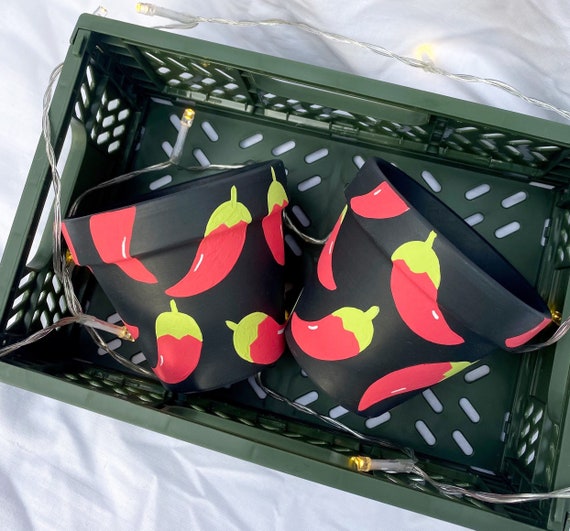In this image, there are two round planting pots, each with an open top and a flat, narrow base, prominently displayed. Both pots are black with vibrant red peppers painted all around their exterior, adding a pop of color and liveliness. The pots are positioned inside a green plastic basket that resembles a milk crate in structure and texture. They appear to be tipped over on their sides rather than standing upright. The basket containing the pots rests on a soft white surface, possibly a sheet or tablecloth, which serves as a neutral background that draws attention to the vivid details of the pots. The image contains no text, allowing the visual elements to speak for themselves.